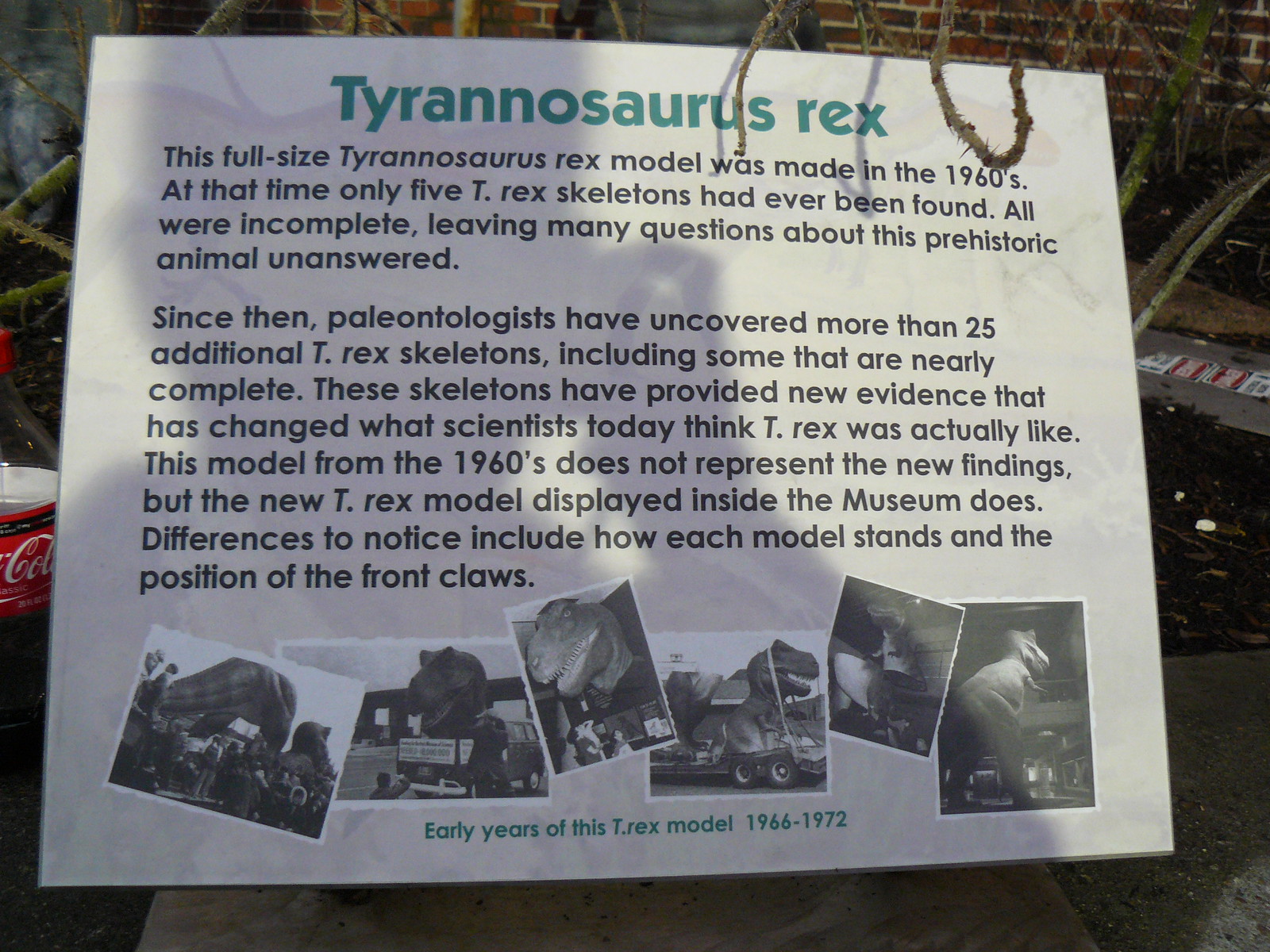This outdoor museum display features an informational plaque titled "Tyrannosaurus Rex" in large greenish-blue letters, accompanied by a shadow image of a T-Rex. Beneath the title, two explanatory paragraphs provide historical context and scientific updates. The first paragraph explains that the full-size T-Rex model, created in the 1960s, was based on incomplete skeletal findings, as at that time, only five T-Rex skeletons had been discovered. The second paragraph details that since the 1960s, over 25 additional T-Rex skeletons—some nearly complete—have been unearthed, offering new insights that have reshaped our understanding of this prehistoric predator. The display notes that while the 1960s model does not reflect these newer discoveries, an updated T-Rex model inside the museum does. Key differences include the stance and front claw positions. The plaque is further adorned with six black-and-white photographs of the early years of the T-Rex model, labeled "Early Years of the T-Rex Model, 1966-1972."